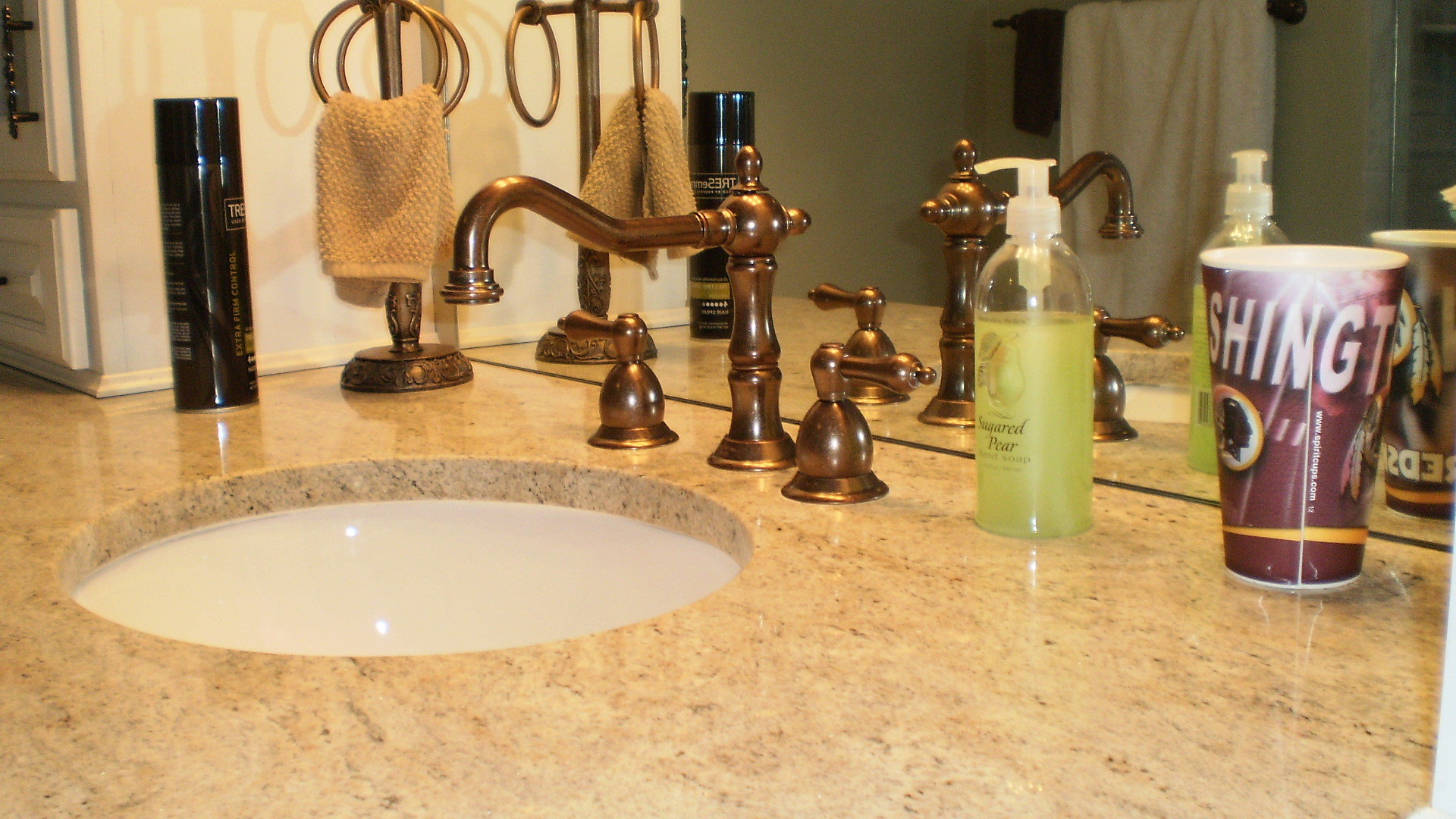The image showcases an elegant bathroom sink with a high-quality appearance. The sink features a lustrous marble countertop in a light orangish-tan color interspersed with brown veining. The centerpiece is a round cutout for the sink basin. The fixtures, including the water spout that arches gracefully before bending downward, are finished in a rich, bronze hue. There are separate faucet handles for hot and cold water.

Complementing the sink is a matching bronze stand adorned with several rings designed to hold hand towels and washcloths. Currently, it holds a brownish-colored towel. Behind the sink, a full-length mirror stretches from where the sink meets the wall, reflecting the entire scene back into the room.

Several items are visible on the countertop. To the side, there's a spray jar of hairspray and a green soap dispenser labeled "Softsoap," though the exact wording is partially obscured. Additionally, there is a purple drink cup with white lettering spelling “SHINGT,” likely referring to "Washington," and it features the profile image of a Native American, suggesting it is memorabilia from the Washington Redskins football team.